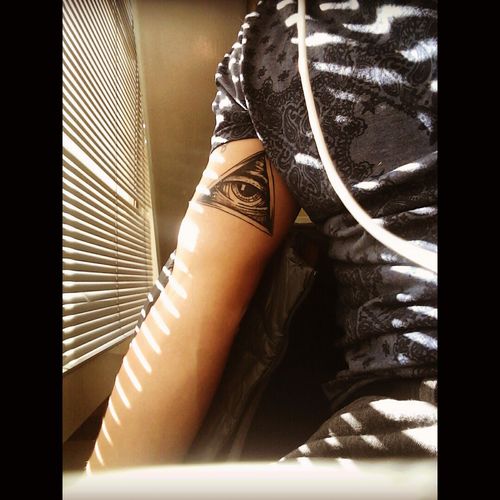In the image, the right side of a man's torso is prominently featured against a gray wall. The man is wearing a black short-sleeved T-shirt with a white pattern on it and green pants. His right upper arm bears a distinct tattoo of a pyramid with an eye inside it, reminiscent of the symbol on the U.S. dollar bill. Sunlight filters through the white window blinds with thin slats to the left of him, casting bright white stripes across his arm and the wall behind him. The man is facing away from the camera, positioned in a somewhat darkened room with a tan wall and black borders on both sides of the image.